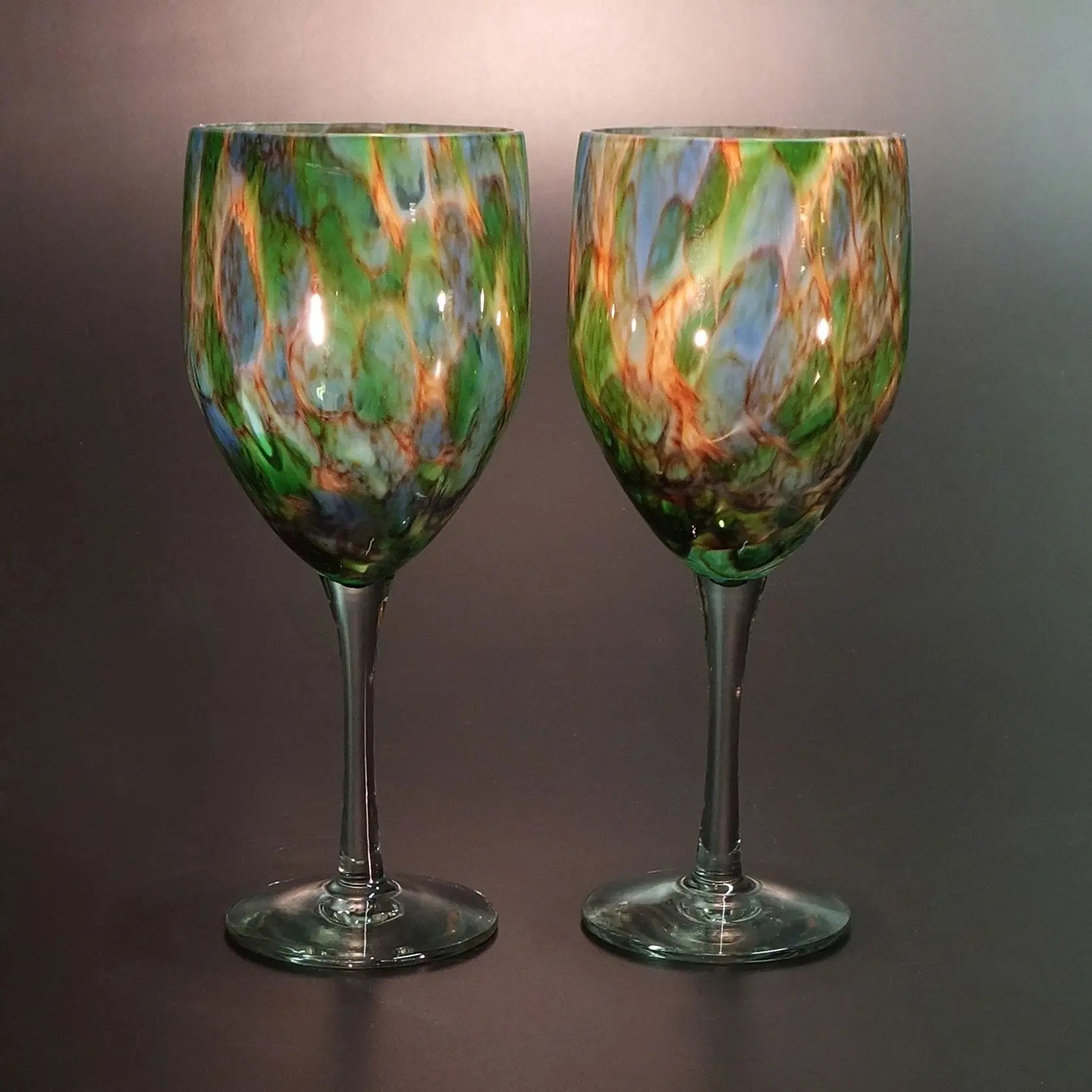This image features two empty, intricately designed wine glasses placed side by side against a plain gray background, with a soft light illuminating the upper part of the glasses. Each glass boasts a long, clear stem and base, while the cup portion exhibits a mesmerizing pearlescent tie-dye pattern of greens, blues, yellows, and oranges. Despite their identical height, each glass's unique, custom-made color pattern ensures no two areas are the same, with variations such as one glass having more prominent greens and the other more blues. Subtle shadows cast by the glasses from the light source enhance the overall professional feel of the photograph.